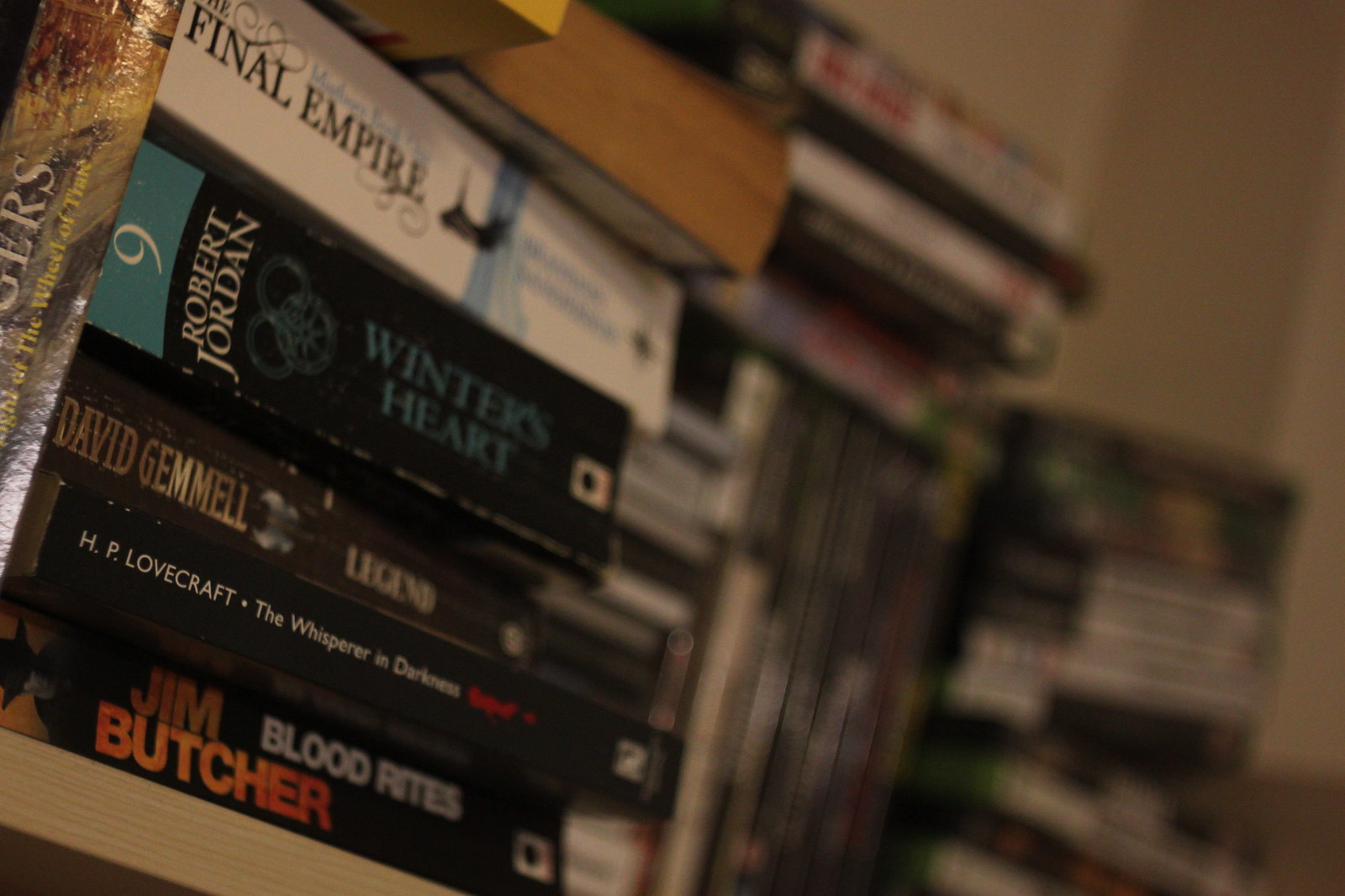In the dimly lit image, a collection of paperback books is piled haphazardly atop a wooden, angled shelf. The stacked books, leaning precariously, create a visually striking foreground. The titles we can discern from top to bottom are "The Final Empire," followed by "Winter's Heart" by Robert Jordan, "Legend" by David Gemmell, "The Whisperer in Darkness" by H.P. Lovecraft, and at the bottom, "Blood Rites" by Jim Butcher. The books predominantly feature black covers, adding to the shadowy ambiance. To the right, the background is blurred, with an indistinguishable stack of books and a potential cabinet discernible only by their vague outlines. The setting is framed against yellow-tan walls, with a possible stereo or additional items below these books, enhancing the sense of clutter and depth. The photographer appears to have utilized the rule of thirds to emphasize the detailed, book-filled foreground.